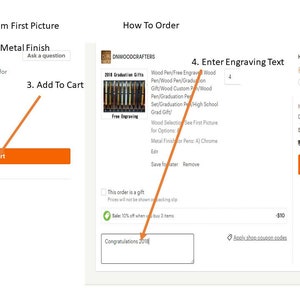This image showcases a screenshot of a shopping app interface. On the left side, partially cut-off black text reads "first picture" against a white background. Beneath this, in bold black text, it states "metal finish." Following that, there is a blurry rectangle with the phrase "ask a question." Below, the word "for" in bold is visible, next to the bolded text and numbers "three dot" and the option "add to cart." An orange arrow points downwards to what appears to be an orange search bar.

In the upper-left corner, the text "how to order" is present above a small image and a set of blurry numbers and letters, likely representing an item number. Towards the right, "number four period enter engraving text" is written. Below, there is an image of pens with blurred text on them; additional blurry gray writing is visible to the right.

Under this section, a statement reads "this order is a gift" with an adjacent checkbox, followed by more indistinct gray text. There's a price tag symbol labeled "safe" and more fuzzy gray writing. Another orange arrow at the top declares "congratulations" accompanied by a number. Adjacent to this is a search bar and additional blurry gray text to the right.